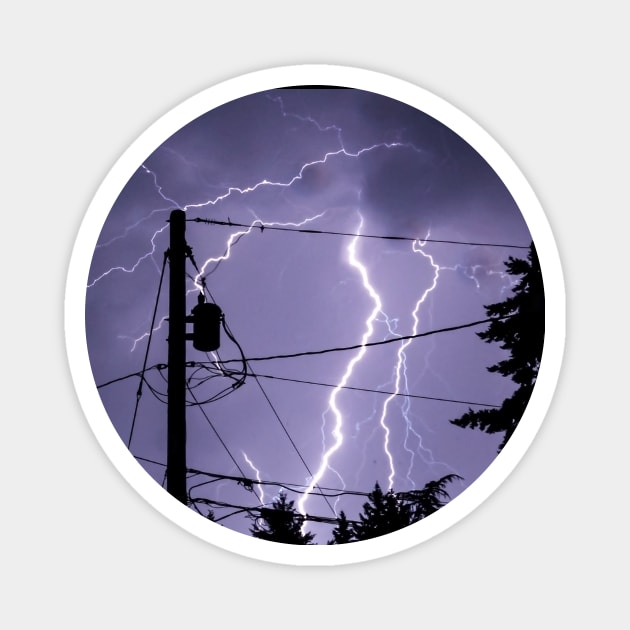The image is a circular photograph with a thick white frame set against a gray background. Within the photograph, a purplish-gray stormy sky dominates, illuminated by multiple lightning bolts crisscrossing the scene. The lightning includes one thinner bolt streaking diagonally from the top right to the left, an upside-down V-shaped pair of bolts also originating from the top right, and a particularly bright, nearly vertical bolt extending from the top right downward. Silhouetted against this electrifying backdrop, a utility pole stands on the left side, adorned with multiple power lines: one extending to the right, two forming a sideways V-shape, and another pair running parallel near the bottom. Attached near the top of the pole is a black cylinder with a nest of wires fanning out, intertwining with the power lines. Encircling the lower and right-hand edges of the frame are the dark silhouettes of evergreen trees, adding a natural contrast to the man-made structures.